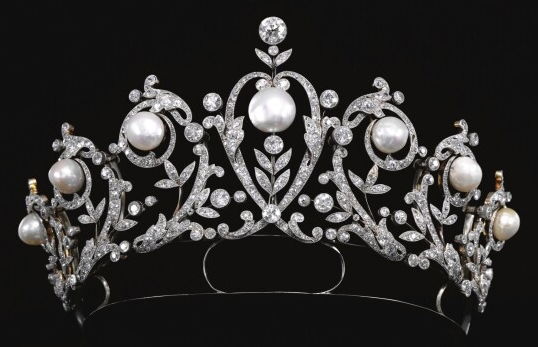The image showcases a delicate white crystal tiara set against a solid black background, emphasizing the intricate details of the jewelry. The tiara features numerous elements made from what appear to be diamonds, forming elegant floral designs and leaf motifs. Central to the design is a heart-shaped diamond, accompanied by additional smaller diamonds that together create a detailed flower, with four leaf-like shapes surrounding a larger round diamond at the top. Enhancing its opulence, the tiara includes a row of seven prominent pearls, gracefully distributed along the middle section of the floral and leaf patterns. The largest of these pearls sits near the top center of the tiara, crowned by a couple of leaf-like diamond structures. The overall design maintains a monochromatic palette, devoid of any dark gold or other colors, ensuring the diamonds and pearls are the focal points. The solid black background serves to further accentuate the brilliance and intricacy of the tiara, making it evident that the photograph aims to highlight the exquisite craftsmanship and elegance of this piece of jewelry.